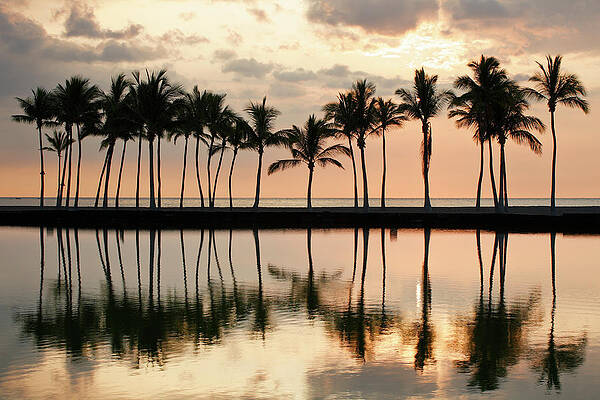This color photograph captures a serene tropical scene at either sunrise or sunset. A narrow strip of land is adorned with tall, slender palm trees, possibly king palms, whose elongated trunks reach skyward. The sky is adorned with puffy clouds, behind which the sun is partially obscured, casting a pinkish or amber hue across the horizon. The photograph beautifully captures the reflection of these majestic palm trees in the calm, slightly rippling water that borders the land on both sides. The tranquil water mirrors the silhouetted trees, while the clouds and the sun create a captivating play of light, making the entire scene appear both vibrant and tranquil. There are no signs of human or animal presence, nor are there any structures or mechanical objects, allowing the pure beauty of the natural landscape to take center stage.